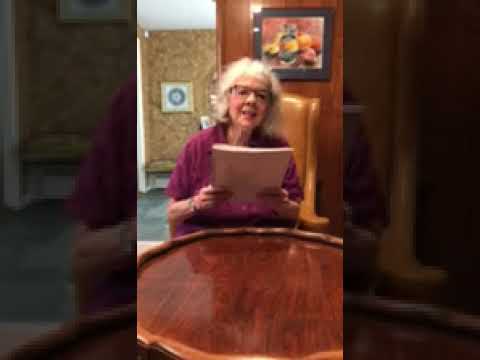The image presents an older woman with shoulder-length, slightly curly white hair, and black glasses, sitting in an orange or brown leather chair. She is positioned behind a small, round wooden table, viewed from the waist up. She wears a dark pink, short-sleeved blouse, and a wristwatch on her right wrist. Her arms are bent at the elbows as she holds what appears to be a stack of papers, a large paperback manual, or a thin magazine. The expression on her face is neutral, possibly mid-speech. Behind her, the wooden wall on the right side features a black-framed painting depicting fruit with a red background. To her left, the room extends into a hallway with lighter brown walls and a white ceiling, adorned with another square picture in a gold frame, showcasing a white background with a dark circle at its center.